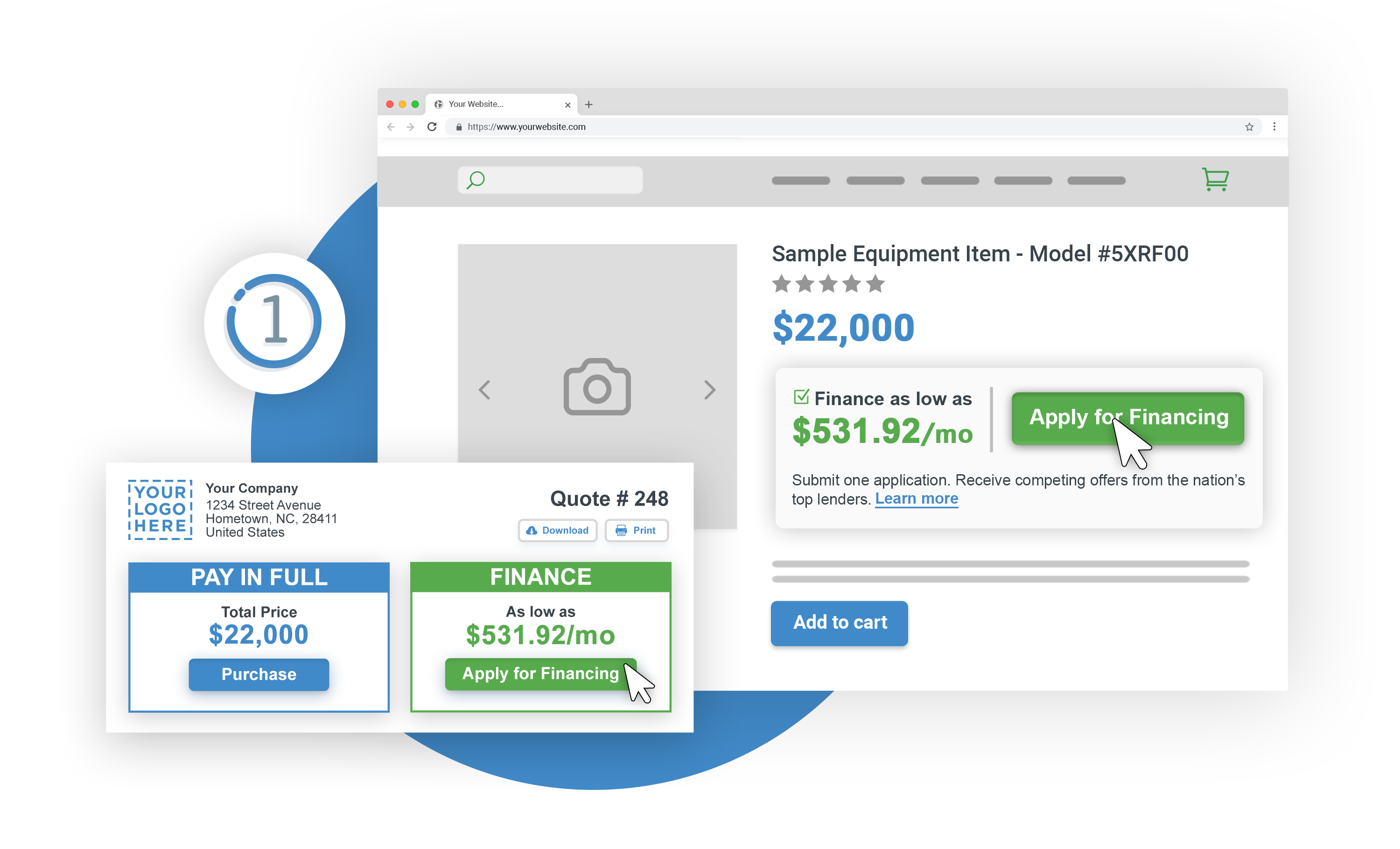The image features a white background with several overlay elements. On the left side, there is a notable blue circle partially covered by these overlays. Adjacent to the blue circle, slightly more to the left, sits a white circle containing a blue line and the number "1" inside it.

In the center of the image, a prominent popup mimics a Mac webpage interface. This popup includes the characteristic red, yellow, and green circles in the top-left corner, typical of Mac OS window controls. Below these, a white tab leads to a gray navigation bar that features a generic search field, simplistic tab indicators, a green shopping cart icon, and a placeholder for a photo. The popup lists a sample equipment model number in black text, with a price of "$22,000" in white. Additionally, it mentions financing options and displays a large white circular cursor, or console, highlighting it.

Overlaying the bottom-left of the image is another page with a white and blue design. It features a placeholder for "Your Logo" at the top, followed by "Your Company Name" in black text, a generic address, and "Quote Number 248." This section prominently displays the payment terms, with "Pay-in-full: $22,000" highlighted in blue and a financing option of "$531.92 per month." A second white cursor is positioned nearby.

The overall composition appears to be a mockup demonstrating how to set up a webpage for financing and payment options for equipment or services.